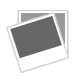This striking advertisement for a magnifying makeup mirror emphasizes its impressive 20 times magnification capability, highlighting its suitability for detailed makeup application and deep facial cleaning. The model featured in the image, a blonde woman with long hair, appears to be in her mid to late twenties and is dressed in a white tank top. She is captured in the act of applying lip gloss to her lips, with a close-up of her lips displayed through the magnifying mirror, making facial pores clearly visible. The circular magnifier, approximately four and a half inches in diameter and housed in a sleek black plastic frame, is depicted as essential for precise makeup application. The ad has a white background, enhancing the focus on the model and the product. Interestingly, a reflection of the model can be seen to the side, further emphasizing the mirror's efficacy. The overall layout of the advertisement, which presents the model prominently with additional details provided below, ensures that viewers understand the product's unique magnification features immediately.